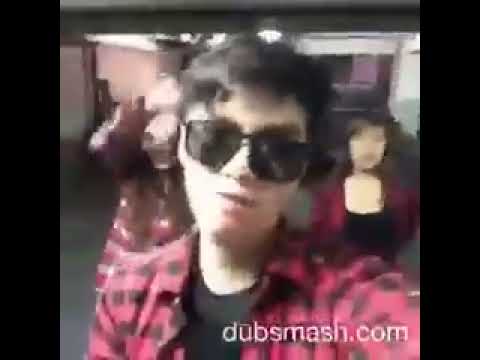The image captures a low-resolution, selfie-style screenshot that appears to be from a commercial or public service announcement, possibly made with Dubsmash. The scene features a young Latino male, approximately 15 or 16 years old, prominently in the center. He's wearing large black sunglasses, a black and red flannel shirt over a black t-shirt, and is holding up a camera to take the selfie. Flanking him are two young women, both slightly blurred and with indistinct facial features due to low resolution. On his right, a young woman with short brown hair, also in black sunglasses and a black and red flannel shirt, tilts her head slightly left, displaying an annoyed expression. Over his left shoulder, another young woman with long brown hair, also dressed in a similar flannel shirt and black undershirt, is visible. The bottom of the image is watermarked with "dubsmash.com," contributing to the quirky and candid nature of this shot where everyone seems engaged in a playful moment, potentially dubbing a song together. The sides of the image are leather-boxed off in black, framing the trio in the center.